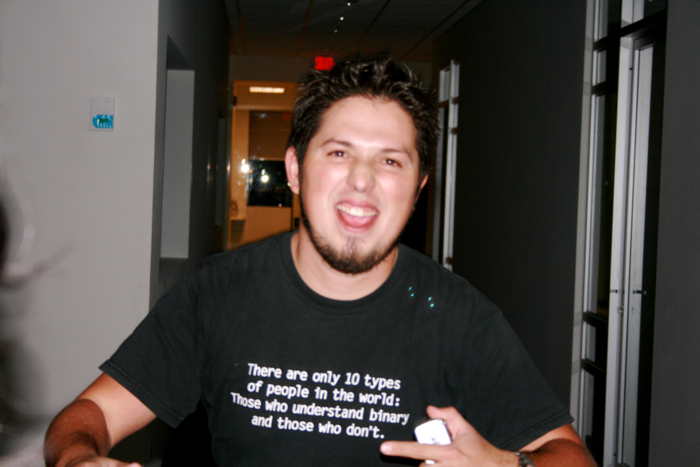The image features a young white man with a trimmed goatee under his chin and short, spiked black hair, likely styled with some product. He is sitting and facing the camera with an energetic, open-faced smile, suggesting he is laughing or enjoying himself at a lively event. He is wearing a black round-neck t-shirt, which prominently displays the quote: "There are only 10 types of people in the world. Those who understand binary and those who don't" in white letters. The young man appears to be pointing toward this quote with one hand, while holding a small white device, possibly a cell phone, in his other hand.

The setting looks like a hallway, dorm, or hotel, with dim and uneven lighting, mainly illuminated by flash, making the background appear darker with some backlighting. Behind him, there's an exit sign and a glimpse of what could be a lobby or a bathroom. On the right side of the image, faint outlines suggest the presence of two window frames, and a white wall with a thermostat is visible in the back-left corner. Additionally, the faint outline of another person's hair is noticeable in the bottom left of the image. The background also includes what seems to be a black TV and some lit rooms, indicating the photo was taken indoors, likely during nighttime. The photograph's overall quality and the reflective flash suggest it could have been taken with a Polaroid or an older camera.